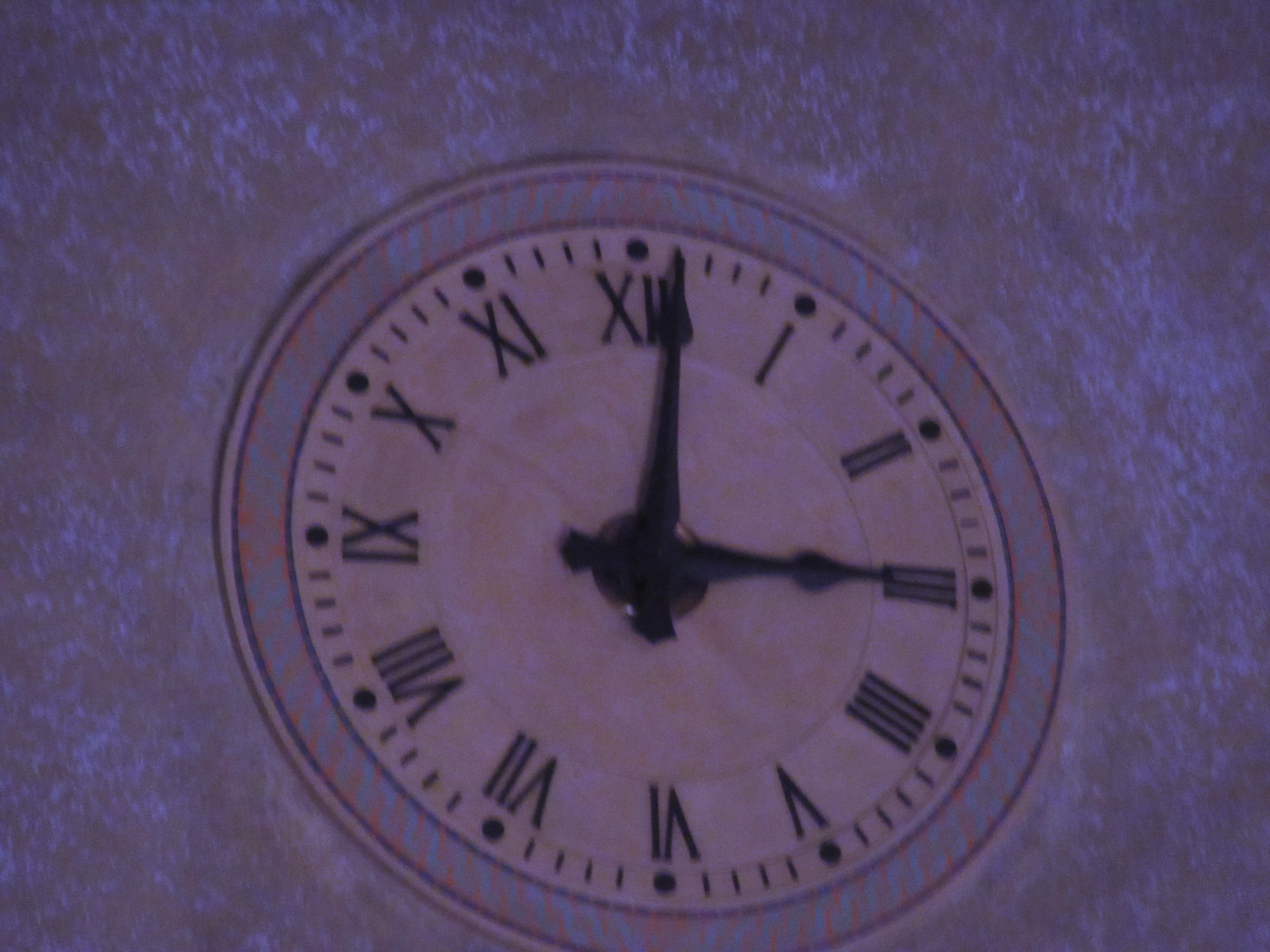The image showcases a prominent, large clock embedded into a wall within a dimly lit room. The clock is illuminated by a soft, diffused light that casts a blue, white, or purplish glow around it, enhancing its presence in the darkened space. The clock features a circular white frame, encasing a pristine white face adorned with black elements for clear readability. The black Roman numerals gracefully encircle the face, marking hours from XII at the top, and progressing clockwise through I, II, III, and so forth, to XI before returning to XII. Black dots, lines, and hands complement the numerals, providing a stark and contrasting visual that emphasizes the clock's classical elegance amidst its modern, ambient setting.